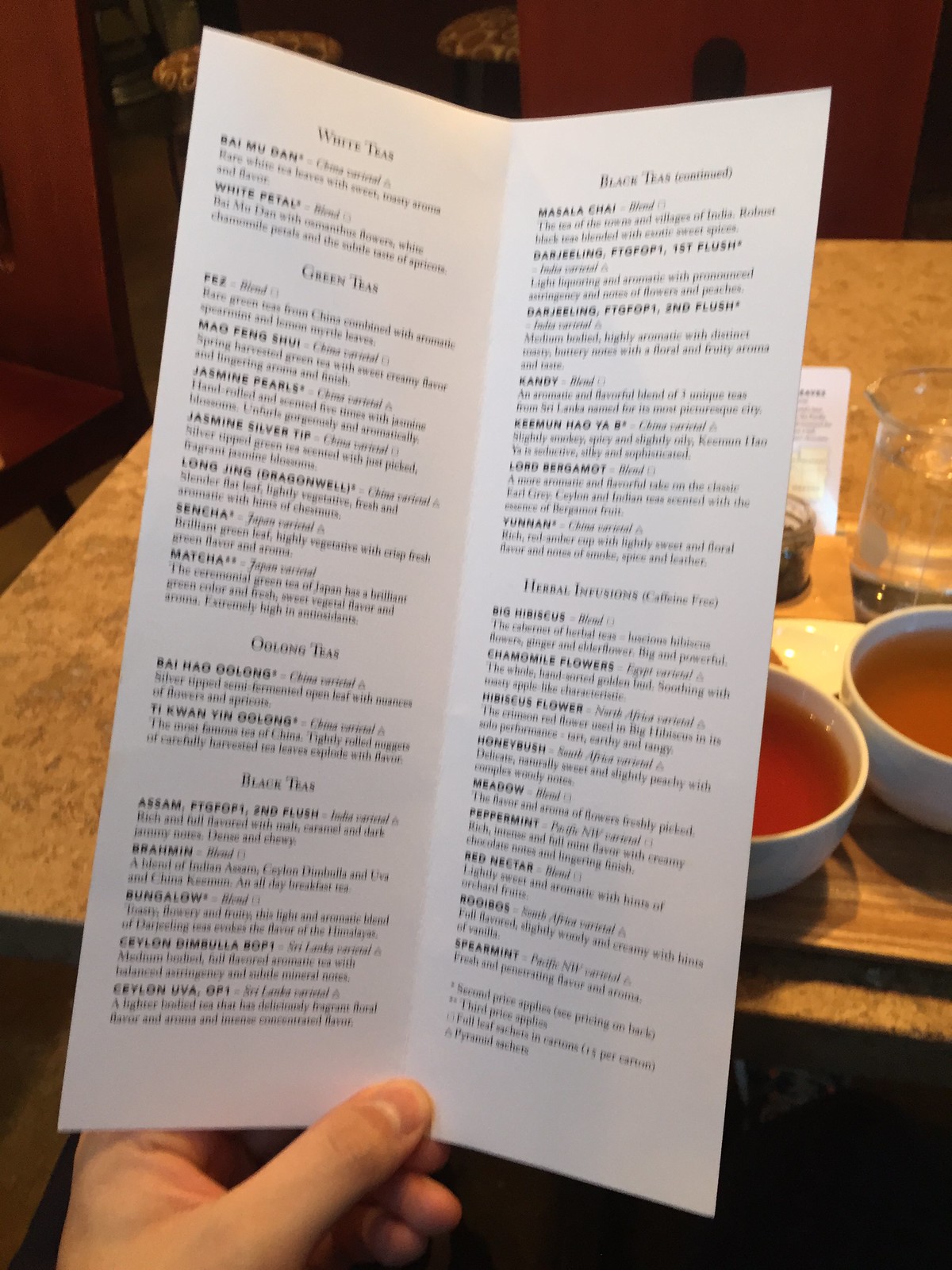This photograph captures a cozy cafe setting, centered around a wooden, patterned table that adds a rustic charm to the ambiance. The table is adorned with a couple of bowls of soup, but no utensils or breadboards are visible, leaving the focus on the table's natural grain and the items on it. Dominating the scene is a person seated at the head of the table, from whose perspective the photo is taken. They are holding a detailed menu featuring an array of specialty teas, including green tea, oolong tea, black tea, and various herbal infusions. The individual's thumb, noticeably pale near the cuticle, holds the menu open, emphasizing the extensive selection of teas. A jug of water is also placed on the table, suggesting a readiness for a relaxing and refreshing experience in this tea-centric cafe.